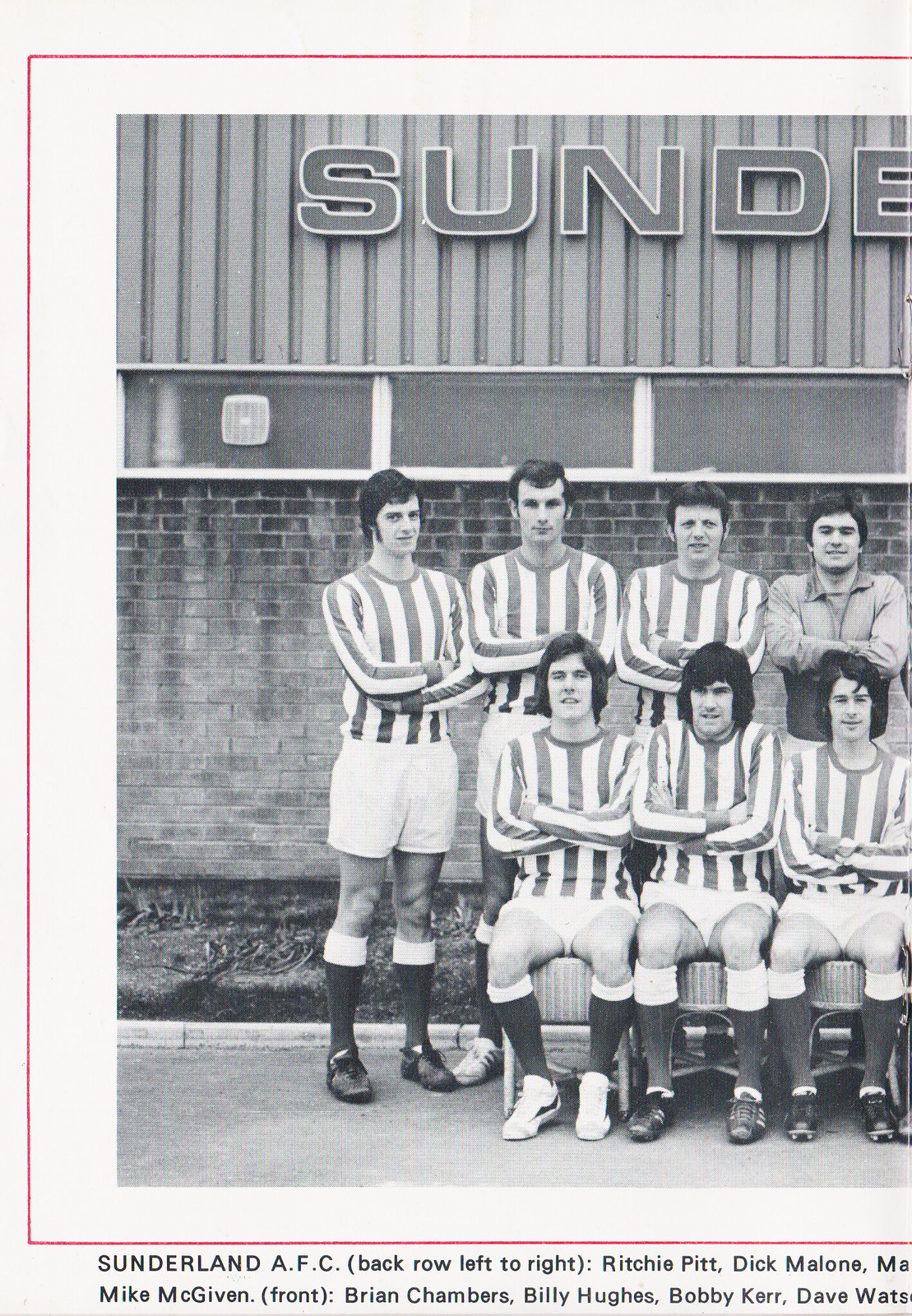This vintage black and white photograph depicts seven young men from a soccer team standing and sitting in front of a brick building with the partially visible letters "S-U-N-D" on its façade. The image is slightly grainy and appears to be cut off on the right side. The players are positioned flush right, with three seated in front, and four standing behind them. They are dressed in vertically striped shirts, white shorts, high black socks with white cuffs, and mostly black shoes, although a few wear white shoes. One individual in the back row to the right is notably not in uniform, opting instead for a button-down shirt. Based on their hairstyles, which suggest a 1970s era, it can be inferred that the photo is several decades old. At the bottom of the image, a caption identifies the team as Sunderland AFC, with names listed for each player: Birchie Pitt, Dick Malone, Mike McGiven (some names cut off), and in the front row, Brian Chambers, Billy Hughes, Bobby Kerr, and Dave Watson. The timeless quality and setting of this image evoke a classic team sports photograph.